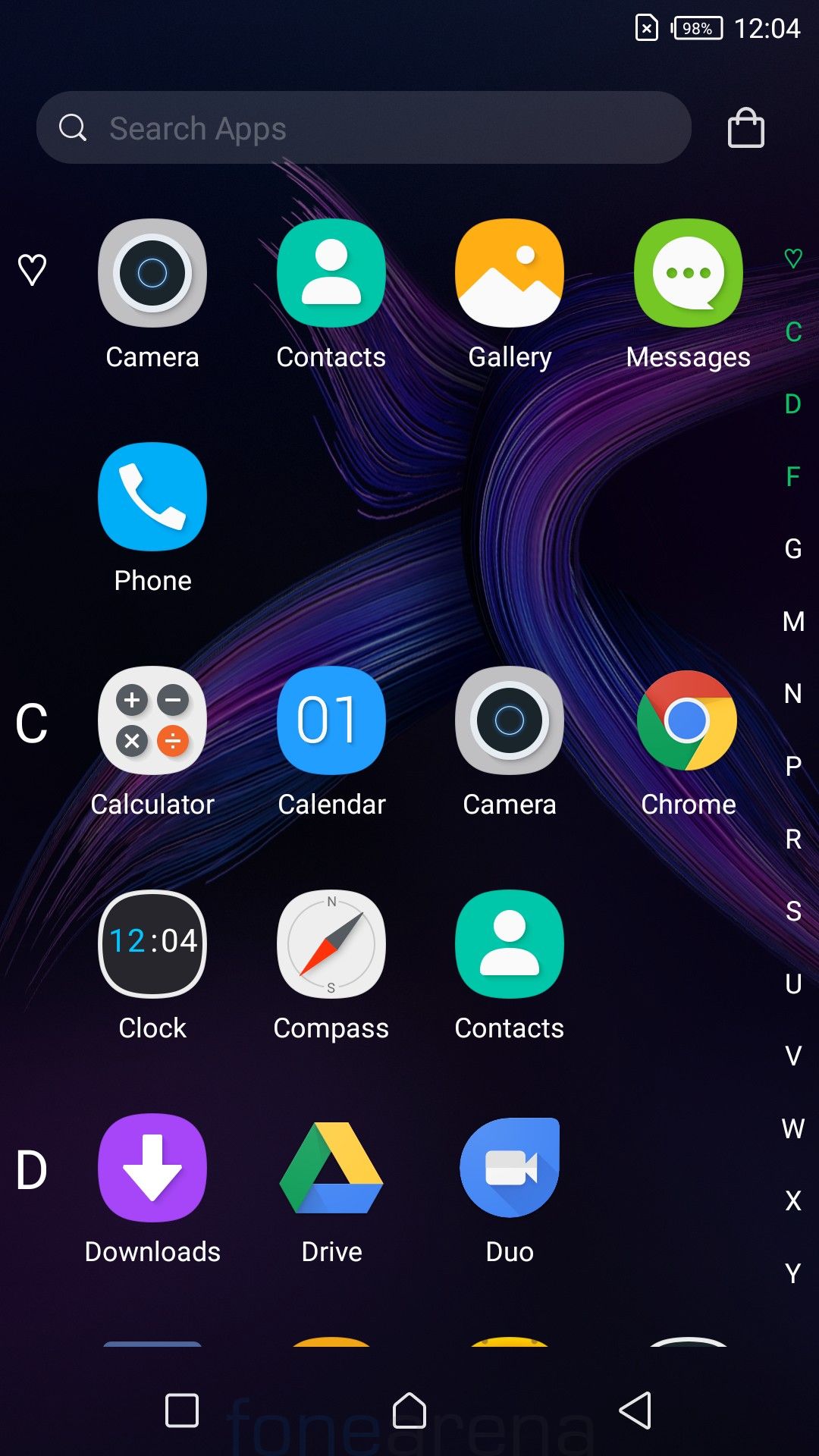This is a screenshot captured from a Google mobile device, as suggested by the multitude of Google applications present. The background is black, and the device's battery is at 98%, with the current time displayed as 12:04. At the top of the screen, there is a search bar accompanied by a small white bag icon. Below the search area, there are several app icons, including a heart icon next to the words Camera, Contacts, Gallery, and Messages, each paired with their respective icons. 

Further down, the screen displays the icon for Phone, followed by a list under the letter "C", comprising Calculator, Calendar, Camera, Chrome, Clock, Compass, and Contacts, each with their corresponding icons. The list continues under the letter "D", showing Downloads, Drive, Duo, and additional icons that are truncated by the screen's lower boundary. 

On the right-hand side of the screen, there is a vertical alphabetical index featuring the letters Heart, C, D, F, G, M, N, P, R, S, U, V, W, X, Y, where the letters Heart, C, D, and F are highlighted in green, indicating the current scrolling position. 

The navigation bar at the bottom of the screen includes three icons: a square for recent apps, a home symbol, and a backwards-pointing triangle for back navigation. The screen captures an interface designed for app navigation, with certain elements cut off due to the screen's limited view.